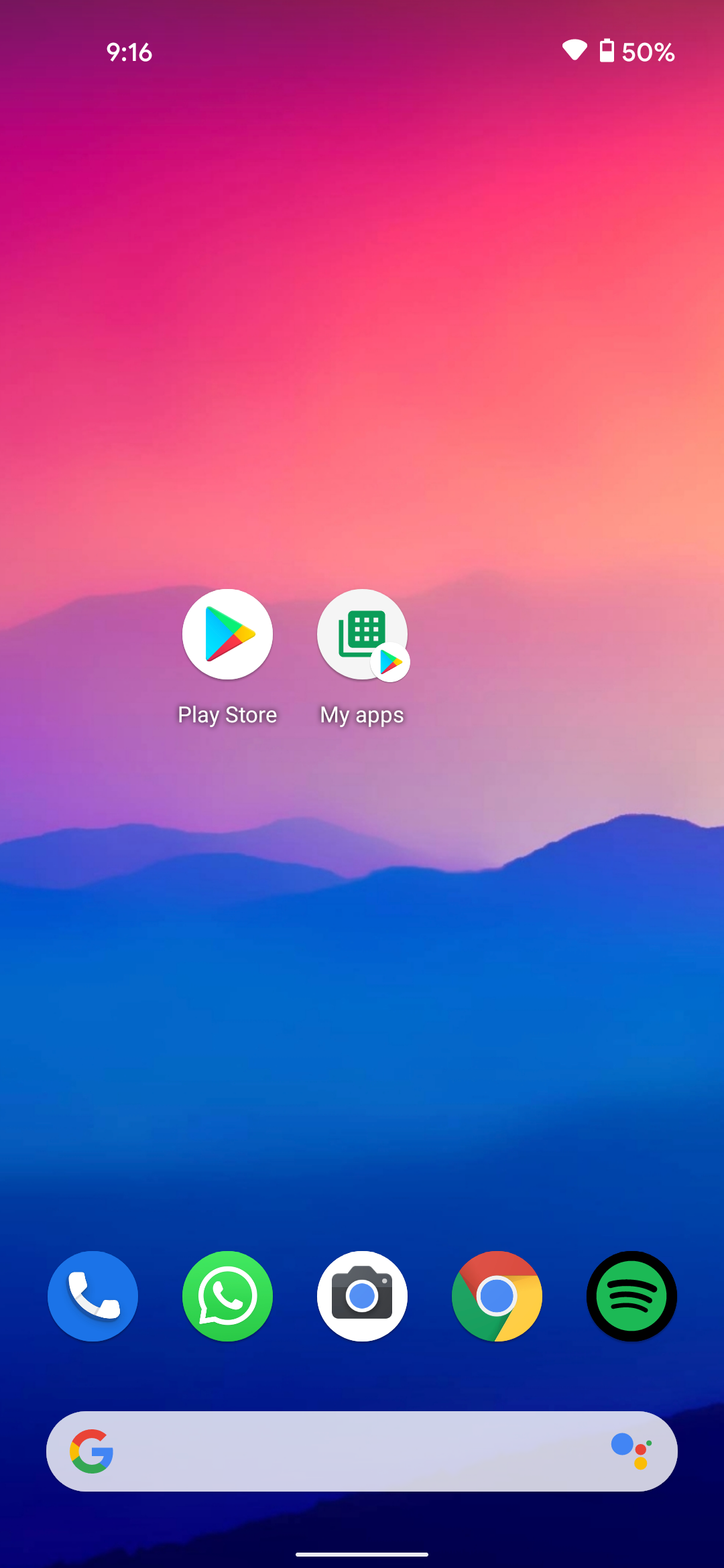The image depicts a smartphone screen adorned with a detailed and artistic background. The time displayed at the top of the screen reads 9:16. To the left of the time, a standard internet strength icon resembling a white baseball diamond is visible. Adjacent to this, on the right side, the phone battery indicator shows it is 50% charged.

Below the status bar, the screen features the Google Play Store icon—a multicolored triangle inside a white button, accompanied by the "My Apps" section symbolized with a green grid-like icon. 

Further down, the dock hosts several essential apps. From left to right, there's a blue phone icon, a green phone icon, a white icon with a camera inside, the Google Chrome browser icon, a Google search button represented with the classic Google logo, and a Spotify logo.

At the bottom of the screen, an empty Google search bar is displayed, prefaced by the colorful 'G' logo for Google.

The background of the phone screen is a visually captivating scene featuring rolling hills painted in a rich blue hue. Above these hills, the sky transitions into a blend of pink and purple tones, creating a dreamy and artistic atmosphere.